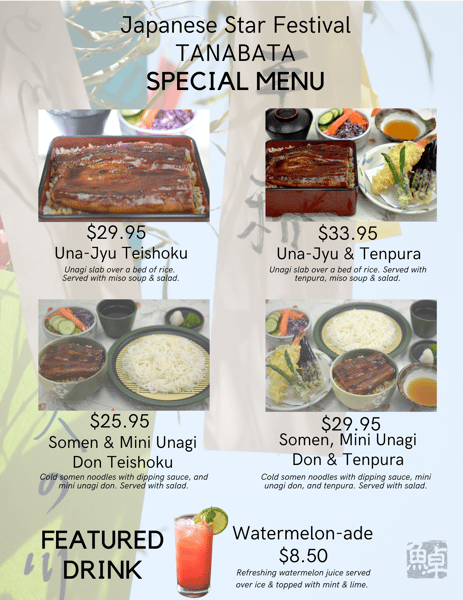The image displays a detailed menu for the Japanese Star Festival, prominently titled "Japanese Star Festival" and "Tanabata" in the center of the upper portion. Beneath that, it states "Special Menu." The menu showcases four main dishes with corresponding prices and descriptions, along with a featured drink at the bottom.

On the left side of the menu, the first dish is Yuna Yu Teishoku for $29.95, described as an unagi slab over a bed of rice, served with miso soup and salad. Below this, the menu features Somen and Mini Unagi Don Teishoku for $25.95, which includes cold somen noodles with dipping sauce and a mini unagi don served with salad.

On the right side, the first dish is Yuna Yu Teishoku with Tempura for $33.95, which is an unagi slab over a bed of rice, served with tempura, miso soup, and salad. Below this, it features Somen, Mini Unagi Don, and Tempura for $29.95, which combines cold somen noodles with dipping sauce, mini unagi don, and tempura, served with salad.

The featured drink at the bottom of the menu is Watermelon Ade for $8.50, described as refreshing watermelon juice served over ice and topped with mint and lime.

Four images accompany the descriptions of the dishes, visually showcasing each meal, and an additional picture represents the featured drink.